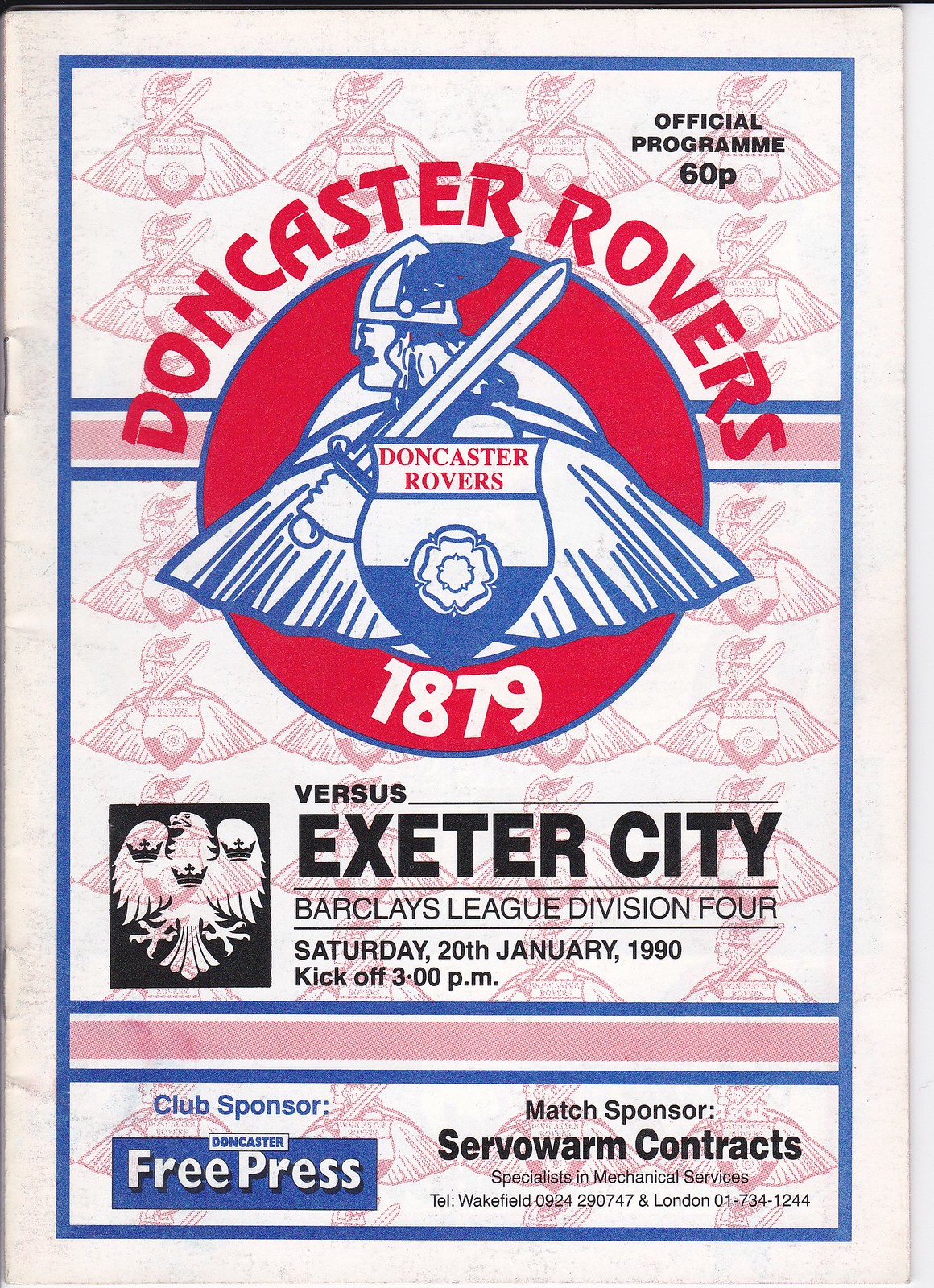The image depicts a well-produced football program for Doncaster Rovers, sized like a regular book page. Dominated by a primarily white background and a blue border, the top section of the program features a red circle emblem with a Viking figure donning a winged helmet, wielding a sword, and holding a shield decorated with a flower. This emblem includes the year "1879" in white text and is repeated in a tile-like pattern in red across the background. The program announces the matchup "Doncaster Rovers vs. Exeter City" in black text, marking the event as part of the Barclays League Division 4. The date and time are specified as "Saturday, 20 January 1990, Kickoff 3 p.m." The top right corner denotes the program's price of "60p". Toward the bottom, sponsorship details are listed: "Club Sponsor: Doncaster Free Press," and "Match Sponsor: Servo Warm Contract Specialists," with contact information for their Wakefield and London offices.